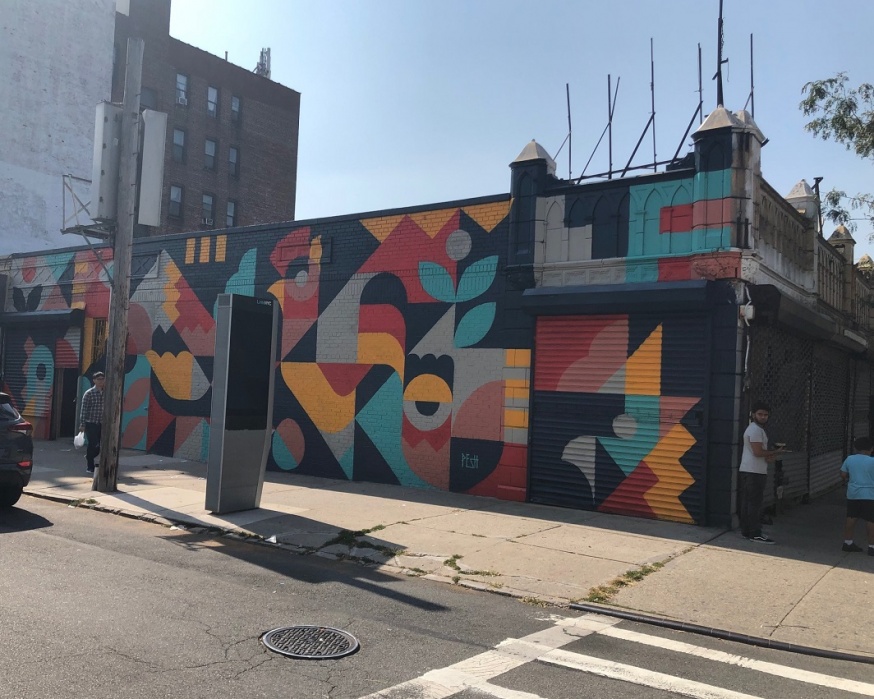This daytime photograph captures a vibrant commercial street scene, dominated by a colorful mural wrapped around the corner of a building. The mural features bold geometric shapes in hues of golden yellow, red, teal blue, and black, evoking intentional graffiti or a professionally designed urban artwork. The building, positioned on the right-hand side, extends horizontally and is bordered by clear blue skies, with the sun gleaming subtly behind another brown building to the left. A sidewalk extends from the bottom right to the mid-left, intersected by a crosswalk that leads from the middle of the image towards the right.

In the foreground, three people animate the scene: a child in a light blue shirt and black shorts with black shoes and white socks stands on the far right, facing away. To his left, a man with long hair, darker skin, attired in a white shirt and black pants, stands next to the vibrantly painted building. Further left, another man, clad in a black and white checkered shirt and black pants and carrying a clear bag, walks towards the child and the other man. On the extreme left, partially out of frame, a black vehicle is parked. Adding to the urban ambiance, a charging kiosk, resembling those found in New York City, stands on the sidewalk, though its operational status is unclear. The background features a tall, multi-story building, contributing to the dynamic urban landscape.